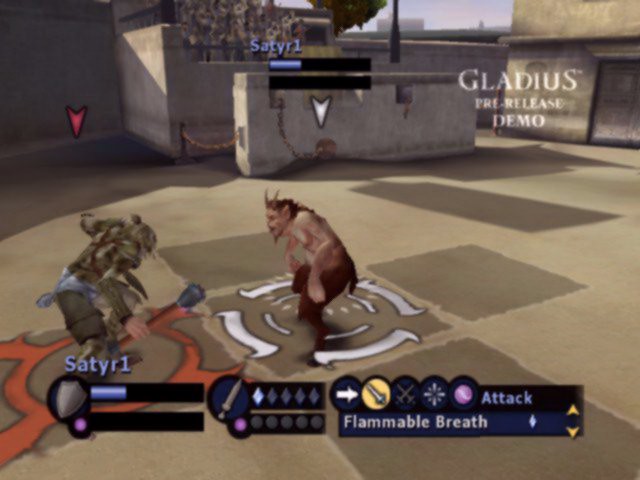A nostalgic screenshot from the classic 1990s or early 2000s computer game "Gladius," specifically from its pre-release demo. The scene takes place in a Roman-themed arena, with two characters poised for combat on a sandy, beige-yellow battleground. On the left, a green-skinned warrior, brandishing a wooden mace with a metal top, crouches ready to strike. Despite their green complexion, the character's hands are skin-colored, adding an intriguing contrast. Opposite the green warrior stands a Satyr—half-man, half-beast—with two prominent horns and a sharp, pointy goatee. The Satyr is bare-chested, with the upper half of its body showing skin, while the lower half resembles that of an animal.

Both characters are highlighted by rings—red around the green warrior and white around the Satyr—indicating their active status in the fight. Behind them looms a stone stand filled with barely visible spectators, reinforcing the arena setting. A smaller stone wall, adorned with a chain, separates the fighting ground from the stand, implying a restricted area.

At the bottom of the screen, a user interface displays vital stats for the Satyr character, including a health bar, a sword icon, and various power and strength indicators. It’s evident that the player controls the Satyr, preparing for a showdown against the green warrior. The detailed environment and interface elements capture the essence of strategic combat in a bygone digital age, encapsulating the game's rich historical ambiance.